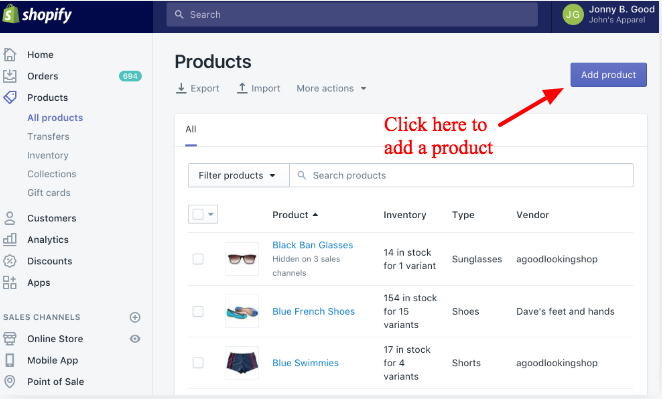The image depicts a detailed screenshot of the Shopify interface, emphasizing various sections and functionalities. At the top, there is a prominent Shopify logo followed by a search bar. A series of green circles labeled "JG" lead to a user account named "Johnny B. Goode" associated with "John's Apparel."

On the left side, a vertical navigation menu lists several options starting from 'Home,' 'Orders,' 'Products,' (which expands into 'All Products,' 'Transfers,' 'Inventory,' 'Collections,' and 'Gift Cards'), followed by 'Customers,' 'Analytics,' 'Discounts,' 'Apps,' and 'Sales Channels.' These channels include 'Online Store,' 'Mobile App,' 'Point of Sale,' and more.

On the right side of the screen, a prominent blue button labeled 'Add Product' is visible, enabling the user to click and add new products. Nearby, filtering and sorting options for products are available, such as filtering by 'Product,' 'Apparel,' 'Inventory,' 'Type,' and 'Vendor.'

The main content area showcases a list of products with details. For example, "Black Band Glasses" are listed as hidden on three sales channels with an inventory of 14 in stock. Another product, "French Shoes," appears with an inventory of 154 and a significant price tag. An additional item, "Blue Sleeves," shows an inventory of 17 across four variants.

The interface is neatly arranged with a clean, grey sidebar to the sides, enhancing the visual appeal and ensuring the focus remains on the central content area.